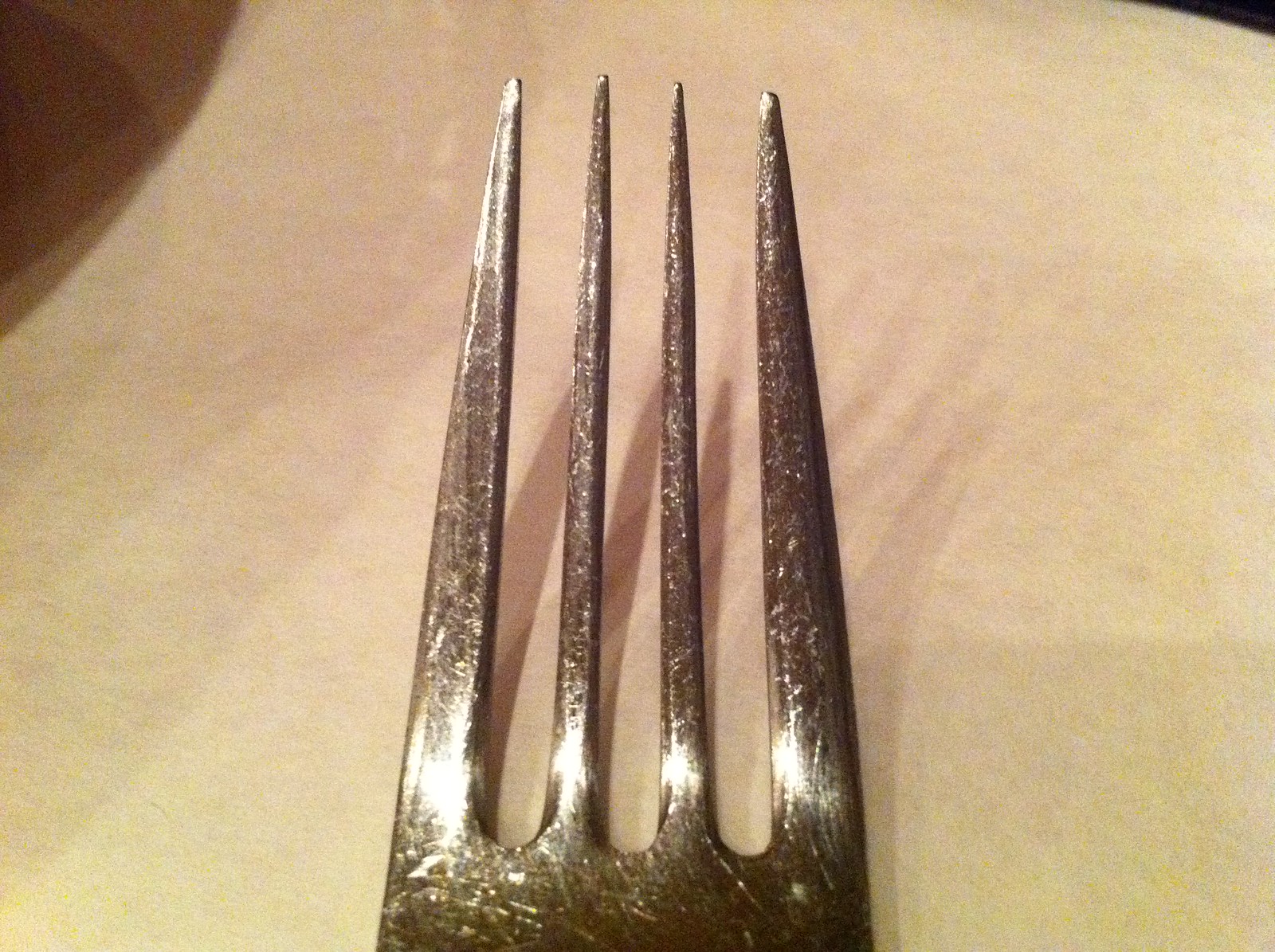This image depicts a close-up of a well-used, scratched, and tarnished fork resting on a beige, slightly textured table surface that might be made of laminate. The most striking feature of this landscape-oriented photograph is the top part of the fork, showcasing its four sharp tines that taper slightly upwards. The two outer tines are wider at their base and narrower at the tip, while the fork overall shows significant signs of wear and tarnish, with varying degrees of brown discoloration and scuffs. Light glints off the fork's surface, casting shadows that suggest multiple light sources from overhead. The upper left corner of the image features a doubled-over shadow, hinting at an object outside the frame, perhaps the photographer's hand or another item. The background is predominantly light beige, with a hint of brown wood visible in the upper-left corner, adding depth to the scene. The fork's reflective chrome or stainless-steel material catches the light, emphasizing its aged and worn condition against the clean, simplistic backdrop.